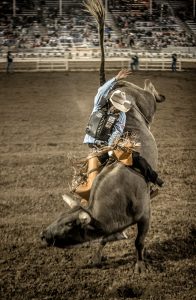The image is a very small, vertically-oriented rectangular photo capturing a dynamic and dramatic rodeo scene. Dominating the frame is a distressed bull, appearing to lose its balance amidst a flurry of activity. Atop the bull, there seem to be two individuals, possibly rodeo participants either attempting to ride or wrestle the animal to the ground. The bull's stance and apparent agitation suggest a struggle of strength and skill. The scene is set within a dirt-filled ring, adding to the authentic atmosphere of a rodeo. In the background, a sturdy fence separates the arena from the stands, which are filled with numerous spectators intently watching the unfolding action. Despite the dim lighting that casts a shadowy ambiance over the image, the energy and tension of the moment are palpable.